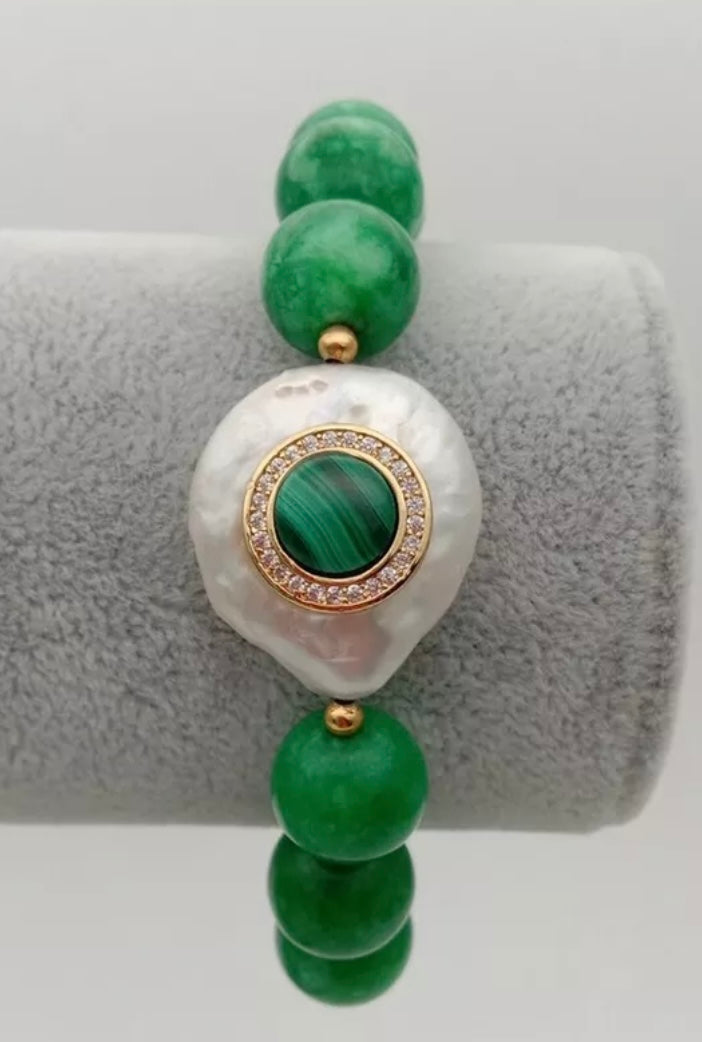The image features a bracelet made of large, smooth, green jade beads, each meticulously spaced with small gold beads. The bracelet is elegantly displayed on a cylindrical padded stand, adorned with a soft, gray fur covering. The centerpiece of this bracelet is a striking jade stone, embedded in a gold circular setting. Surrounding this central jade is an iridescent, pearlesque stone that shimmers like mother-of-pearl. A double gold ring encircles the jade and in the space between these rings, there are clear stones that resemble either diamonds or cubic zirconia, adding an extra touch of brilliance to the piece.